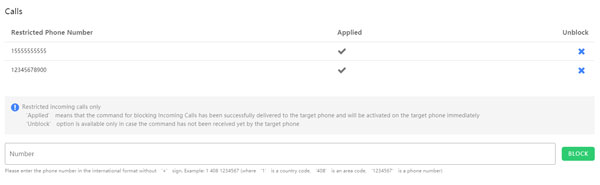A screenshot of a cell phone display shows the call management page with a focus on handling restricted calls. The interface is set against a white background. At the top left, bold text reads "Calls." Below this, three main categories are listed: "Restricted Phone Number," "Applied," and "Unblock."

The first listed phone number is 15555555555. Under "Applied," a black checkmark indicates the blocking command has been successfully delivered and activated on the target phone. Under "Unblock," a blue X is present. A gray dividing line separates this listing from the next.

The second phone number displayed is 12345678900, which similarly shows a black checkmark under "Applied" and a blue X under "Unblock."

An instruction box with a blue circle and exclamation point icon provides an explanation. It reads, "Restricted incoming calls only. 'Applied' means that the command for blocking incoming calls has been successfully delivered to the target phone and will be activated on the target phone immediately. 'Unblock' option is available only in case the command has not been received yet by the target phone."

Below, there is an entry field where users can input a phone number. To the right of this entry field is a green button labeled "Block." The final section provides further instructions, advising, "Please enter the phone number in the international format without a sign, e.g., 14081234567," followed by additional guidelines on entering the correct area code.